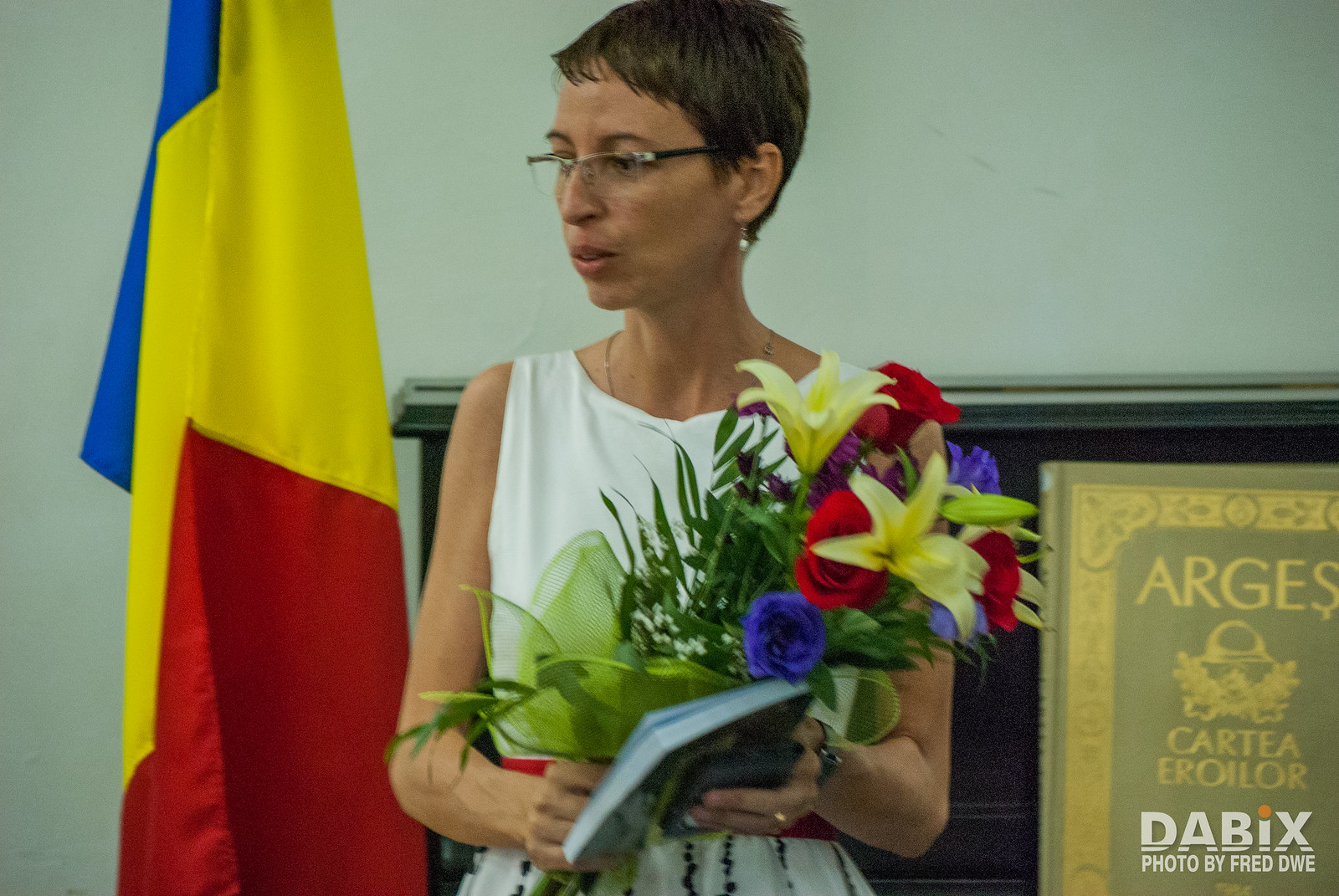In this image, a woman with short brown hair and glasses, featuring thin frames and black arms, is standing center stage, possibly at a celebratory event. She dons a sleeveless white dress adorned with dark vertical stripes at the hem and is accessorized with a pearl white earring in her left ear and a slender necklace. Her mouth is slightly open, as if preparing to speak. She holds a vibrant bouquet of flowers, featuring red, blue, yellow, and purple blooms with prominent green leaves and stems, in her right hand. In her left hand, she's grasping a book and possibly a cell phone. Behind her, a wooden podium is evident, as well as a blue, yellow, and red flag. A sign with the yellow letters "A-R-G-E-S" and additional text, including "Cartier" and "Dabeck's photo by Fred Dewey," is visible against a dark background. The scene includes a white wall, and a black countertop can be seen over her shoulders.